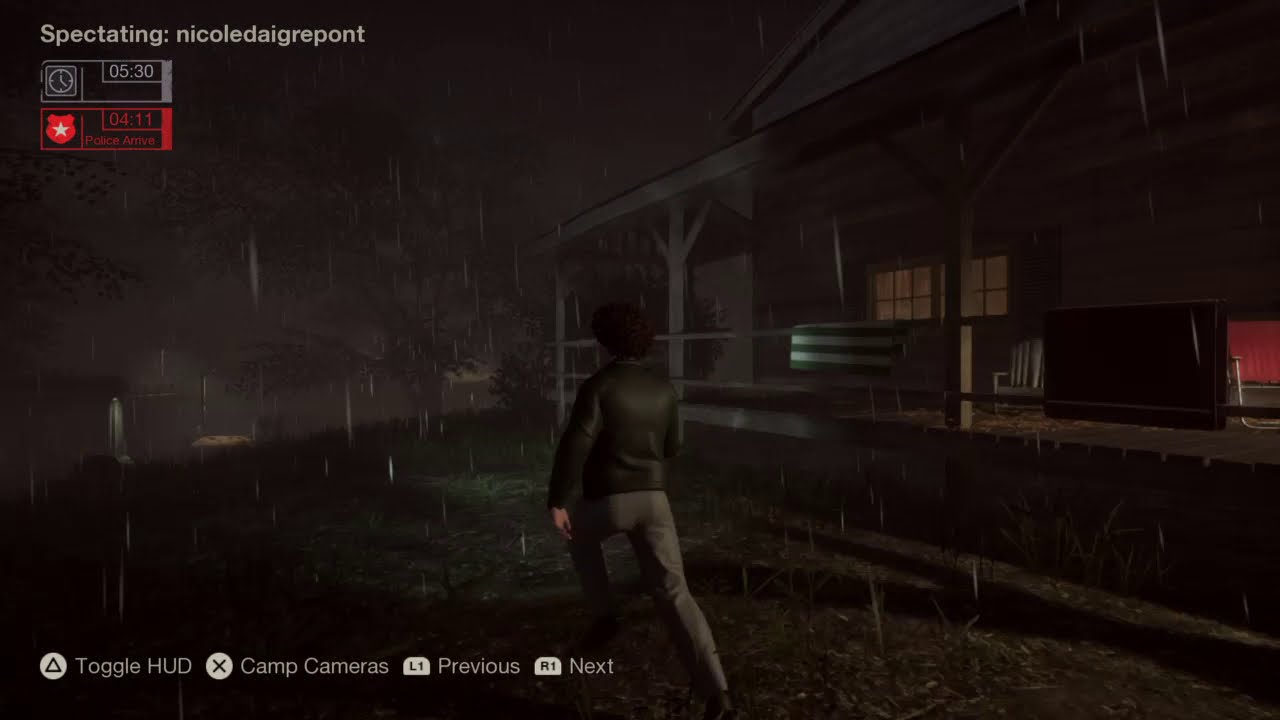This is a highly detailed full-color digital image from a video game, captured during a nighttime rainstorm. The scene is horizontally rectangular and portrays an atmospheric outdoor setting. At the top left, the screen displays the text "Spectating: Nicole Diagri-Pont," and at the bottom, there are instructions for the player on the use of their hand controller, including options to toggle the HUD, swap cameras, and navigate between different views.

The central element of the image is a figure seen from the back, possibly jogging or walking briskly. The individual's gender is indiscernible. They are dressed in a green or black jacket and gray or darker tan pants, with dark hair and a visible Caucasian hand. The figure is moving to the left of the frame, in front of what appears to be a large cabin or farmhouse characterized by wooden planks and a covered porch that wraps around the structure. This porch includes several chairs, suggesting a residential setting.

Further details enhance the moody ambiance: the ground consists of grass and dirt, and the horizon on the left side of the image fades into a foggy, spooky area dotted with trees, adding to the eerie atmosphere of the night. Overall, the image vividly captures the immersive environment of the game with meticulous attention to rain-soaked detail and a sense of movement and purpose from the central character.